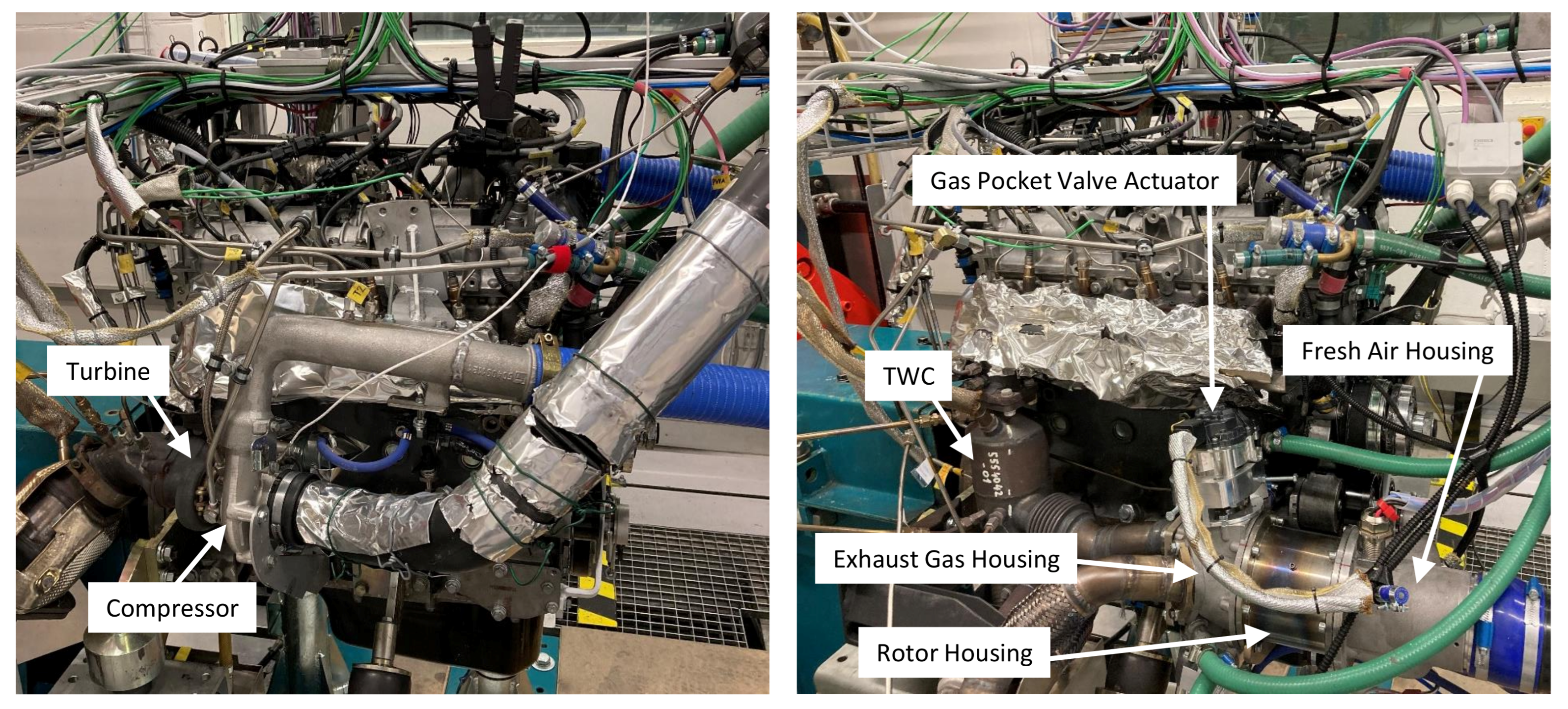The image features two side-by-side color photographs of intricate machinery, possibly a component of a heating or air conditioning unit. Each photograph, square in shape, is labeled with white rectangular boxes containing black text and white arrows pointing to various parts.

In the left photograph, a complex assembly of gray metal, silver piping, and numerous dangling wires is visible. Among the components, the labels identify a "turbine" and a "compressor." A prominent silver pipe, resembling a dryer vent, is also noted, along with a multitude of smaller tubes and pipelines.

The right photograph showcases the same machinery from a different angle, again highlighting the intricate network of hoses, tubes, and wires. This image features multiple labels pointing to specific components: "gas pocket valve actuator," "fresh air housing," "TWC," "exhaust gas housing," and "rotor housing." The machinery's complexity is underscored by the various gaskets and attachments visible throughout the image. The color palette across both photographs includes black, white, gray, silver, green, blue, teal, yellow, red, copper, and purple, enhancing the detailed technical illustration of the unit.